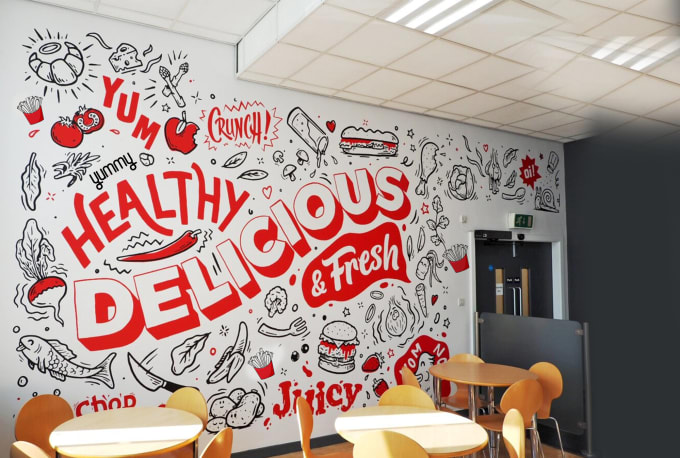The photograph captures the interior of a restaurant in landscape format, focusing on a large, white side wall adorned with numerous food-themed murals and lively text. Dominating the wall are black and white illustrations of various food items including croissants, leaves, fish, bananas, potatoes, broccoli, onions, and chicken drumsticks. Interspersed among these are red-themed images such as tomatoes, apples, beets, hot dogs, ketchup, strawberries, and a radish. The wall also features vibrant red text in various playful fonts and styles with words like "yum," "crunch," "healthy," "delicious," "fresh," "yummy," and "juicy" scattered throughout. At the forefront of the image are three simple, light brown wooden dining tables, each surrounded by four matching chairs. The ceiling, visible in the shot, is white with a square pattern and fitted with luminescent lights. Additionally, a black double door and an adjacent black wall are noticeable on the right-hand side of the image. The overall scene exudes a casual, welcoming atmosphere with a focus on wholesome and delicious food.